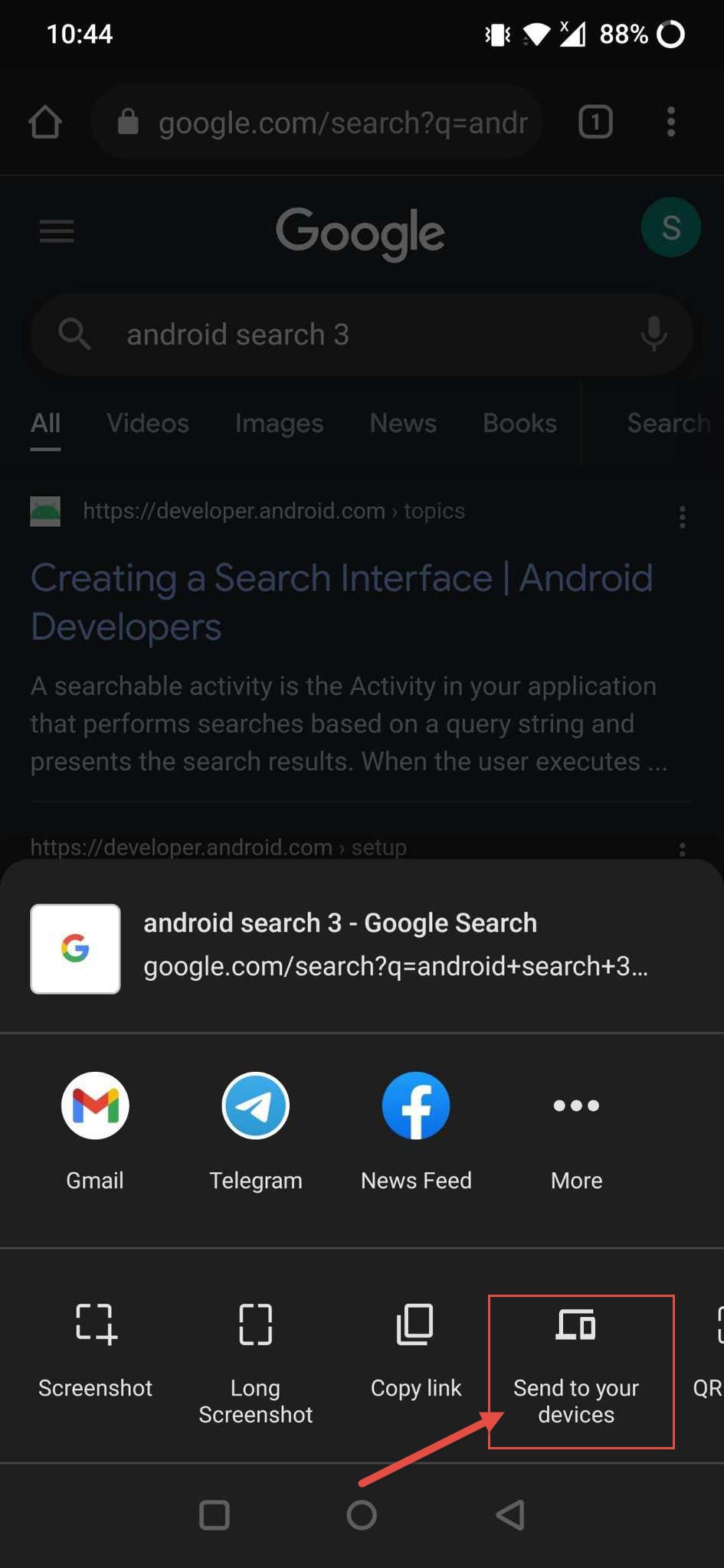This is a detailed and cleaned-up caption for the provided screenshot:

---

The image is a screenshot from a cell phone, taken at 10:44 with an 88% battery level. The screenshot displays a Google search results page for the query "Android search 3." The search result in focus is titled "Creating a Search Interface | Android Developers" from the official Android Developers website, which is accessible via URL: https://developer.android.com. The description underneath the title outlines that a searchable activity in an application performs searches based on a query string and presents the results upon user execution.

Additionally, multiple notable icons are present:
- The Gmail logo, characterized by its multi-colored design (blue, red, yellow, and green) forming an 'M' shape within a white circle.
- The Telegram logo.
- The Facebook logo, recognizable by its blue and white 'F' emblem.

A red arrow is prominently pointing towards a "Send to your devices" option. There are also three dots, indicating a menu option, positioned both at the top right corner of the screen and next to the main search result.

---